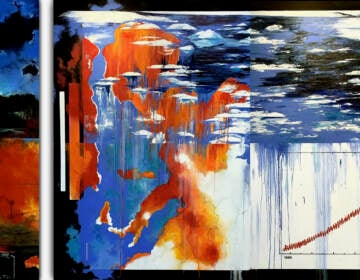This color photograph captures an abstract painting with a dynamic and textural composition. Predominantly featuring white, light purple, blue, black, and orange tones, the artwork blends these colors in various ways. The top section of the painting is characterized by a mottled mix of blue, black, and white hues, creating a sky-like effect. This section appears to be dripping down into the white area below with thin, deliberate lines, resembling rain. Towards the left center near the bottom, a prominent splotch of light purple houses an orange mass that forms the distinct shape of a boot with an upturned, elf-like heel. Adjacent to this, an orange area is made up of jagged lines, injecting vibrant energy into the lower part of the piece.

On the left-hand side, there's a straight vertical white bar that runs from the top to the bottom of the painting, accompanied by black vertical bars above and below it which are tinged with purple and white. Furthermore, beyond this white bar, red blotches intermingle with blue sections. These blotches extend down, mingling with the blue drips over the white portion, giving an impression of varied layers and depths. Accompanying this central motif, the leftmost edge of the painting features an orange and blue mass. The overall composition is brought together by a squiggly brown line inside a black box that appears to rise on the right. Although no discernible objects, people, or animals appear, the piece evokes nature elements through its color dynamics and forms.